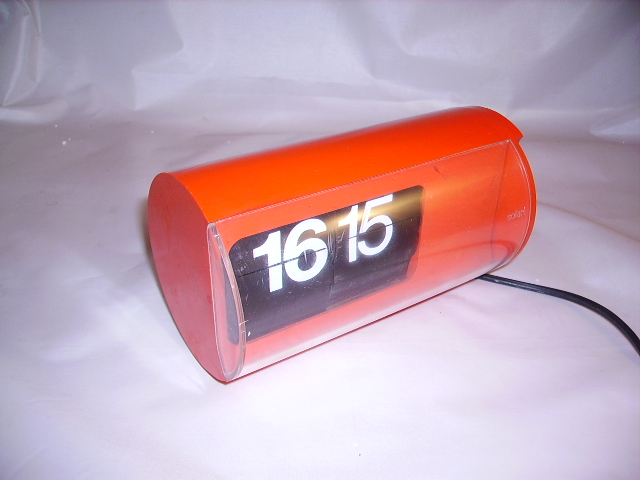The image features a unique, retro-style alarm clock reminiscent of the pneumatic tube systems used in banks for secure transactions. The clock is horizontally positioned, revealing a red rear casing that houses its functional components. The front display is enclosed by a clear, circular cover with flat ends, giving it a distinctive cylindrical appearance. A black power cord extends from the clock, while the screen prominently displays the time "16:15" in military format. The word "solar" is visible on the front, possibly indicating solar-powered functionality. The alarm clock is showcased against a clean, white background, suggesting a studio photography setting.